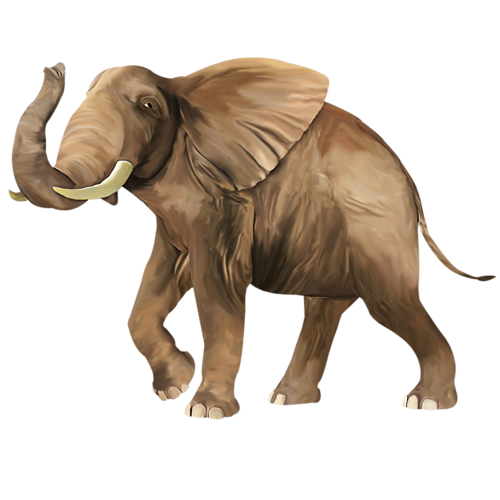This is a detailed, artistic rendering of a brown elephant set against a white background. The elephant is facing towards the left side of the image with its trunk raised upwards to forehead level, giving it an imposing and dynamic posture. Both of its white tusks are visible, though partially obscured at different angles due to the raised trunk. The right front leg of the elephant is bent at the knee, hovering off the ground as if the elephant is in the midst of taking a step. The full body is displayed, revealing a large, detailed form with the legs spread slightly apart, and a narrow tail at the rear. The color palette primarily consists of various shades of brown, with darker shadows on the legs and under the torso, and lighter, tannish highlights on the face, trunk, ear fronts, and hindquarters. The painting incorporates contrast and shading, giving the image depth and dimension, particularly around the legs and left side of the face. The elephant's left ear is visible, appearing to swing back, adding to the sense of movement and life in this vivid hand-painted artwork.